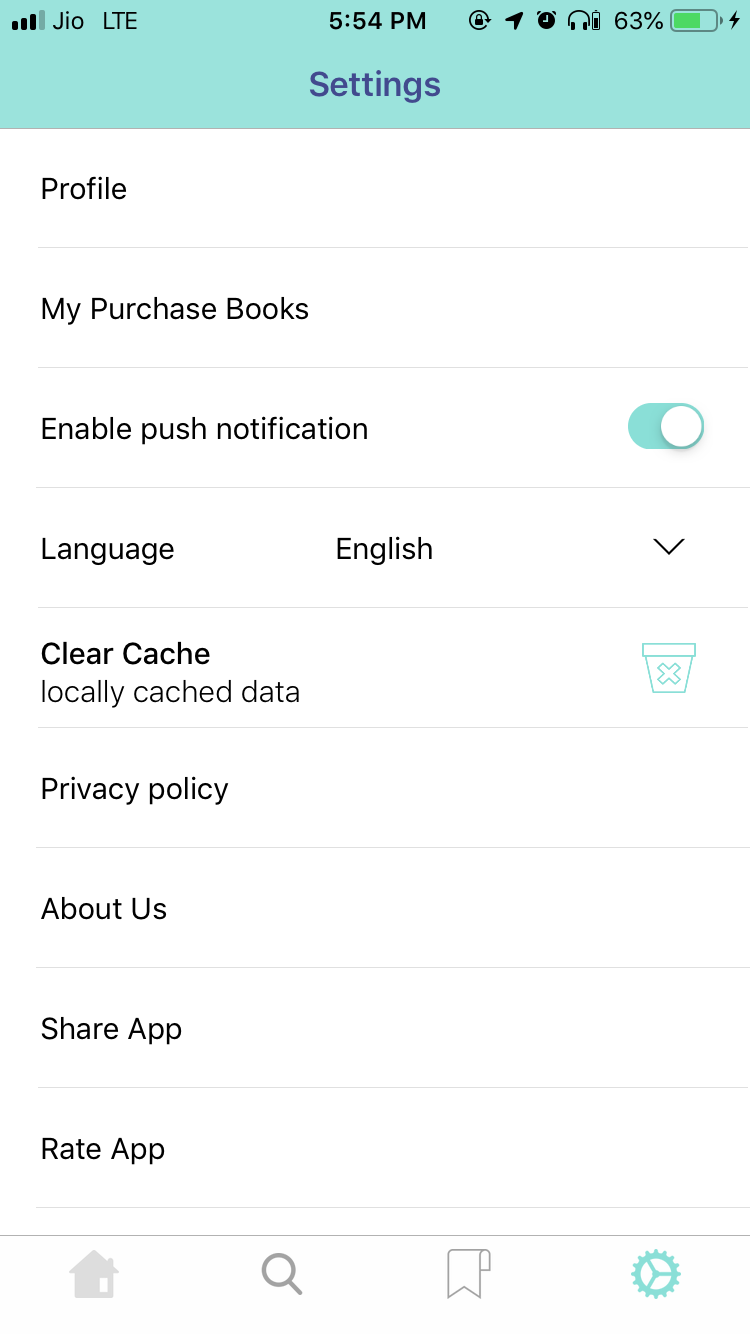The image is a vertical screenshot from a smartphone, captured against a plain white background. At the top of the screen, the status bar is visible with several indicators: the signal strength bars in the upper left corner, followed by the carrier name "JIO" in black text next to the LTE icon. Centered in the status bar is the current time displayed as "5:54 PM" in black. On the right side, a collection of icons is present, including headphones, a clock, and a locked padlock symbol. The battery icon is illuminated green, showing a 63% charge and indicating that the phone is currently charging.

Below the status bar, the central part of the image features a setting menu with various options. The background color of this section is a subtle sage or mint green. Listed down in black text are the following options: 

- Profile
- My Purchase Books
- Enable Push Notifications (with the toggle switch turned on)
- Language: English
- Clear Cache (with a trash can icon next to it)
- Privacy Policy
- About Us
- Share App
- Rate App

At the very bottom, there is a navigation bar with icons colored in teal. These include a house icon, a magnifying glass for search, a ribbon, and a settings button, which is currently highlighted.